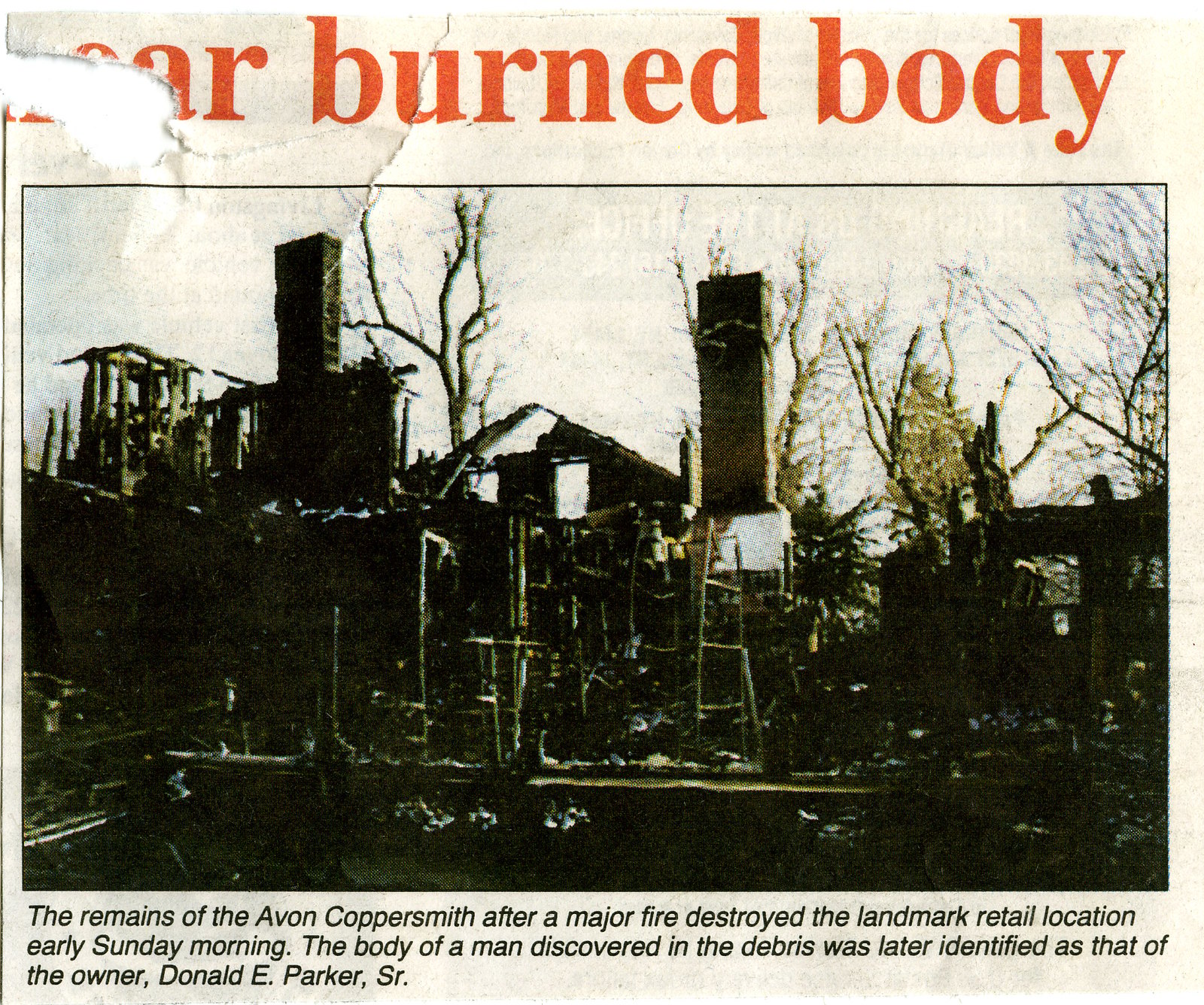The image is a black-and-white photograph showing the aftermath of a devastating fire. At the top of the image, partially torn text in large, red-orange font reads "BURNED BODY." The main focus of the photo is a burned-out building, possibly a house, with charred wooden framework scattered about and chimneys standing intact in the upper left and center right areas. The caption beneath the image, in black text on a white background, provides details: "The remains of the Avon Coppersmith after a major fire destroyed the landmark retail location early Sunday morning. The body of a man discovered in the debris was later identified as that of the owner, Donald E. Parker, Sr." The photograph captures the extensive destruction caused by the fire, highlighting the collapsed portions of the structure amidst the rubble.